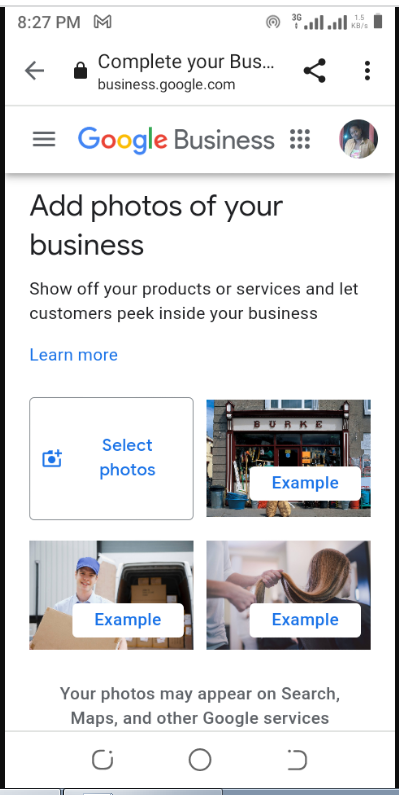Screenshot of a webpage from business.google.com prompting users to add photos for their business. At the top of the page, there's a header titled "Complete Your Business Profile" accompanied by an image of a woman, likely an African American, though her features are not clearly visible. Below this header, there’s a section encouraging users to "Add Photos of Your Business" with the purpose of showcasing products or services and giving customers a glimpse inside the business. This section offers a "Learn More" link for additional information.

Further down, there are four boxes. The first box, currently blank, displays an icon of a camera with the prompt "Select Your Photo." The next three boxes contain example photos: the first one depicts a storefront, the second shows a van with a man holding a package, and the third features a woman getting her hair styled, showcasing long, beautiful hair. An informational note at the bottom mentions that photos added may appear on Google Search, Maps, and other Google services.